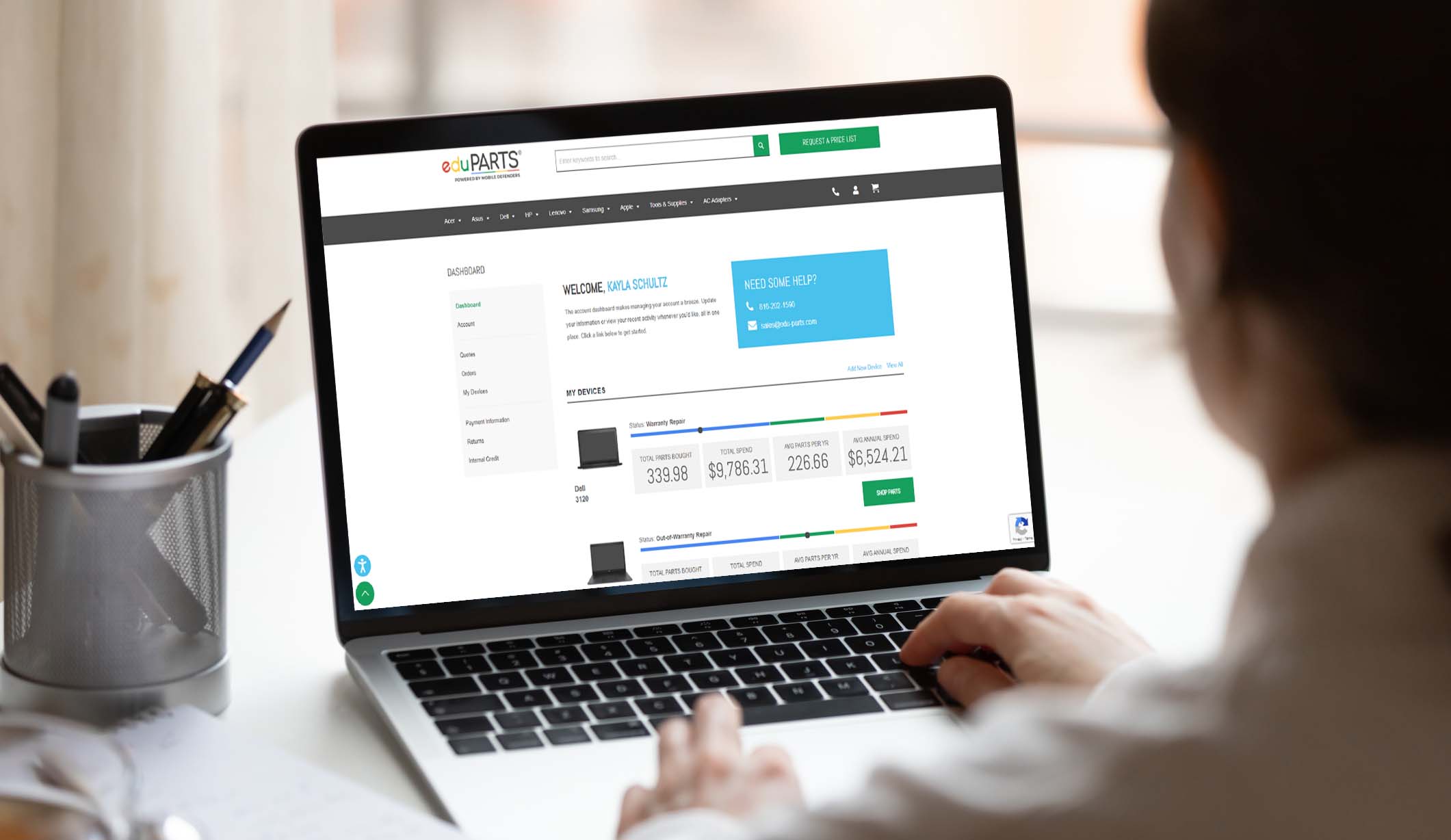The image depicts an advertisement featuring a young individual of European descent seated at a desk, typing on a laptop computer. The person is wearing a white garment, which could be either a shirt or a blouse. To the left of the laptop, there is a pencil cup.

On the laptop screen, the displayed website is 'EDU Parts.' The website's interface includes a search bar at the top, followed by a black navigation bar with nine tabs, each featuring drop-down arrows. To the right of these tabs, there are icons for phone contact, user account, and shopping cart.

Within the main body of the website, a greeting reads "Welcome Carla Schultz." Adjacent to this greeting on the right side is a box that reads "Need some help?" accompanied by phone and mail icons. Further down, there are options labeled "Preferences."

The screen also shows two laptop images, each with a colored bar indicating a range of prices for parts. The bars transition from blue on the left to green, yellow, and finally red on the right, suggesting a gradient scale for pricing.